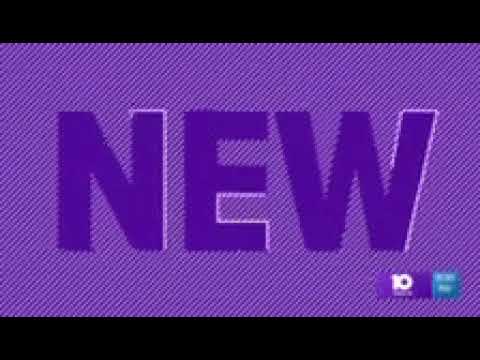The image is a still from a live television broadcast, capturing a minimalist yet distinct scene. Dominating the center of the image is the word "NEW" in prominent purple letters, each with incomplete white borders. The background behind this central word is a purple field composed of parallel, obliquely angled lines, creating a textured, almost static-like pattern. In the bottom right-hand corner, there is a small, rectangular panel typical of news station logos. This panel features the number 10 on the left side of an elongated purple box, with what appears to be the station's call letters beneath. To the right of this, a fuzzy blue or green square contains white text that is illegible due to the low resolution of the image. The overall setup suggests a simple, possibly low-resolution screen grab from a television news broadcast, highlighted by the purple-themed text and background.